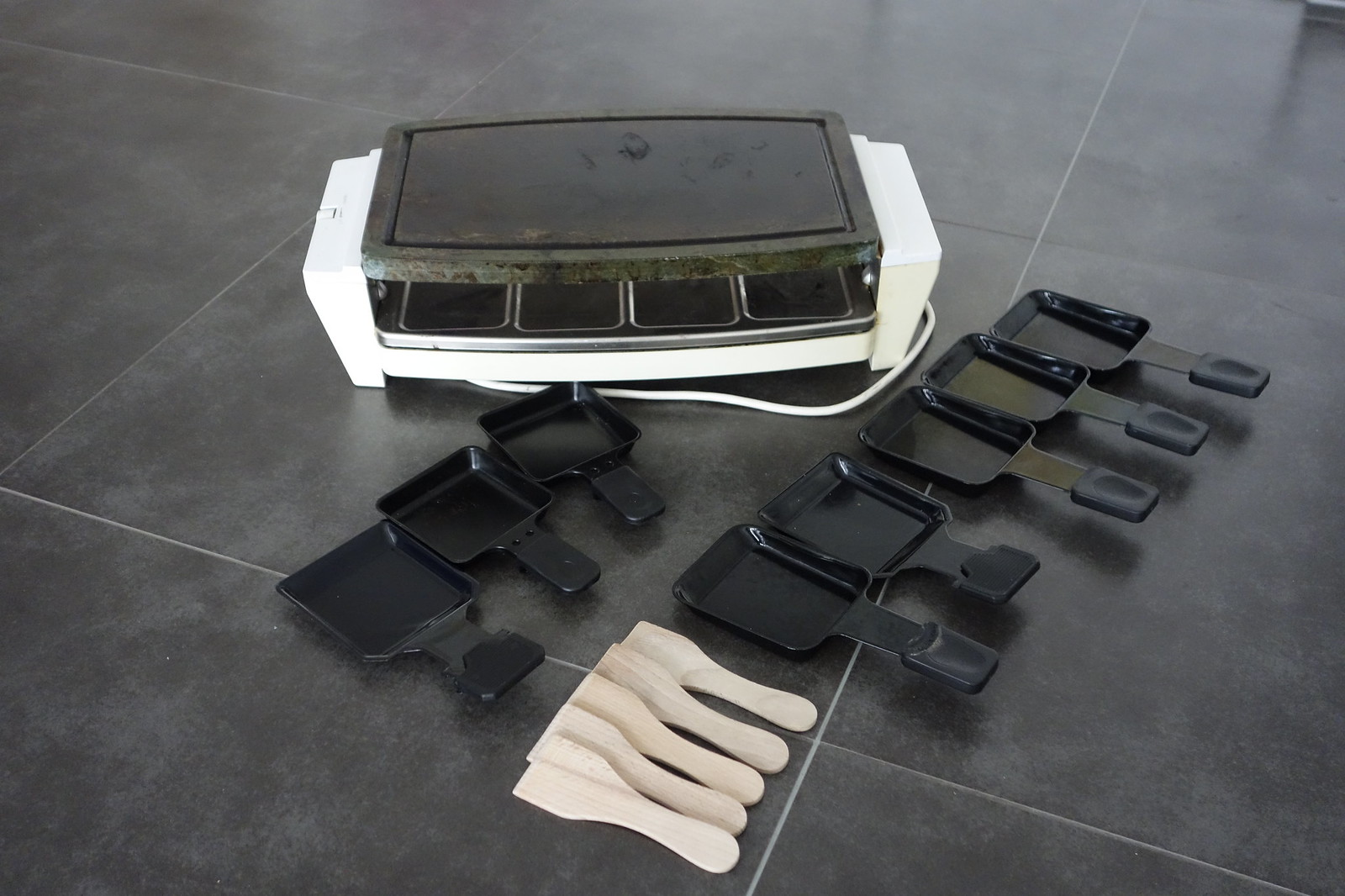This photograph presents a well-lit, rectangular image of a dark brown and black tiled floor with white grout. Centrally positioned on the floor is a small, white electric griddle with a black cooking surface, which appears dirty with splotches of black and green. The griddle’s white cord is neatly tucked underneath the appliance. In front of the griddle, various components are laid out: three square, scooped oil collectors with small rectangular handles—one of which is gray and bent upwards. Adjacent to these are four additional trays of similar design. To the right of the griddle, there are six beige, wooden scrapers arranged neatly. The collective setup suggests a detailed scene of kitchen equipment prepared for use or cleaning.